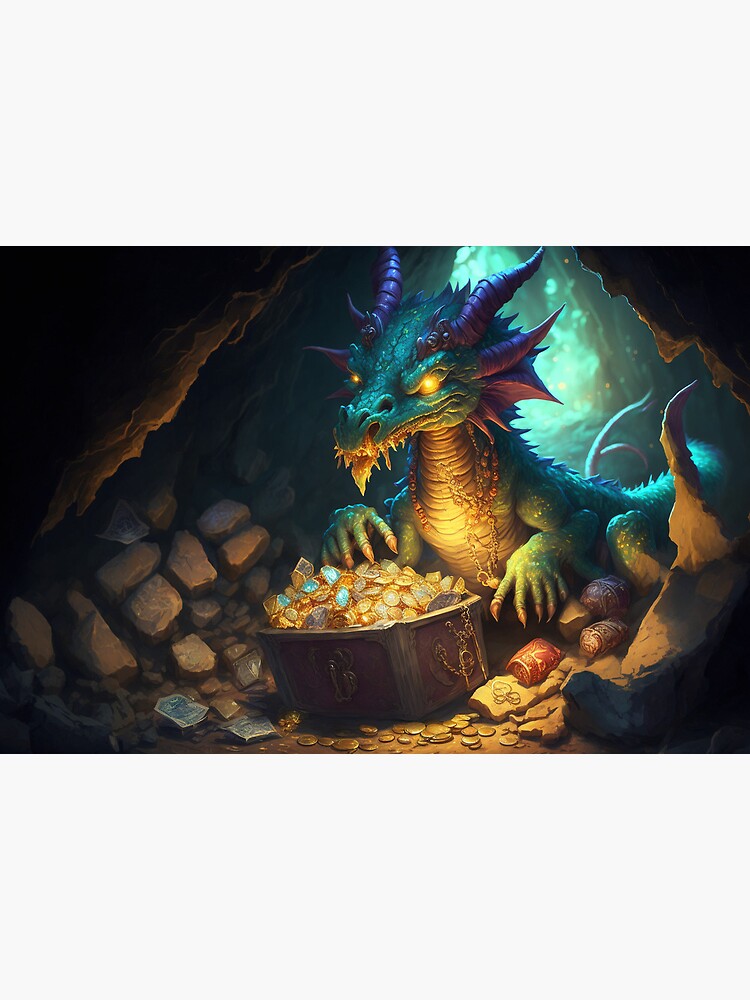This is an intricately detailed illustration of a fantasy dragon guarding a luminous treasure chest within a dimly lit cave. The dragon, predominantly green with turquoise shades, showcases a menacing appearance complete with tentacle-like appendages sprouting from its jaw and neck area. It boasts multiple rippled horns shaded in blue and purple, progressively decreasing in size down its head, and possesses formidable claws with orange nails. The dragon’s fiery, glowing eyes add to its menacing look.

The scene is illuminated by a mysterious greenish-blue aqua light emanating from behind the dragon, casting an eerie glow within the cave. In front of the dragon sits a treasure chest brimming with glowing gold coins, jewels, gems, and rings, with the dragon’s hand resting protectively on the treasure. Surrounding the chest are boulders and rocks, and scattered nearby are valuable vase-like objects and playing cards.

The dragon is depicted in a stance that reflects its protective nature over the treasure, its detailed fingers and digits emphasizing its formidable presence against the backdrop of the dark, rocky cave.